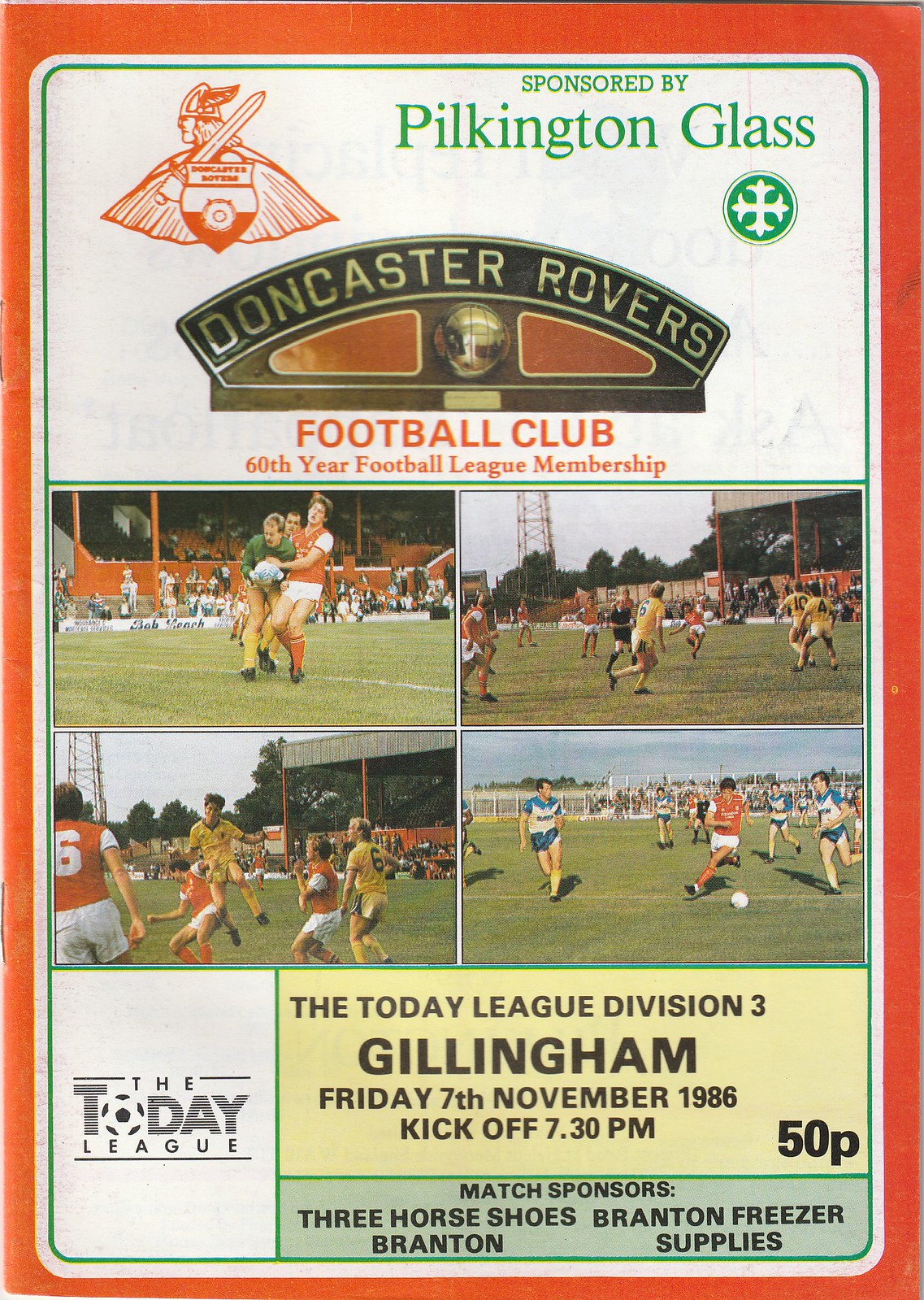This vintage advertisement features a red frame surrounding a vibrant poster celebrating the 60th year of the Doncaster Rovers Football Club’s membership in the football league. At the top left corner, the club logo is prominently displayed, featuring a figure with a conical hat with wings, wielding a sword and shield, adorned with ‘Doncaster Rovers’. The top right corner highlights the primary sponsor, Pilkington Glass, with its green circular emblem housing a white cross.

The centerpiece of the poster comprises four photographs arranged in a quadrant, showcasing the various youth teams in action, dressed in red and yellow kits, reflecting the club's spirited performances. Below the images, detailed match information is provided -- “The Today League Division III,” “Gillingham,” and the event date, “Friday, 7th November 1986,” with kick-off scheduled for 7:30 PM, and entry priced at 50 pence. The match's sponsorship is generously supported by 'Three Horseshoes Branton' and 'Branton Freezer Supplies.’ The blend of nostalgic aesthetics and meticulous detailing encapsulates the historic essence of Doncaster Rovers Football Club.